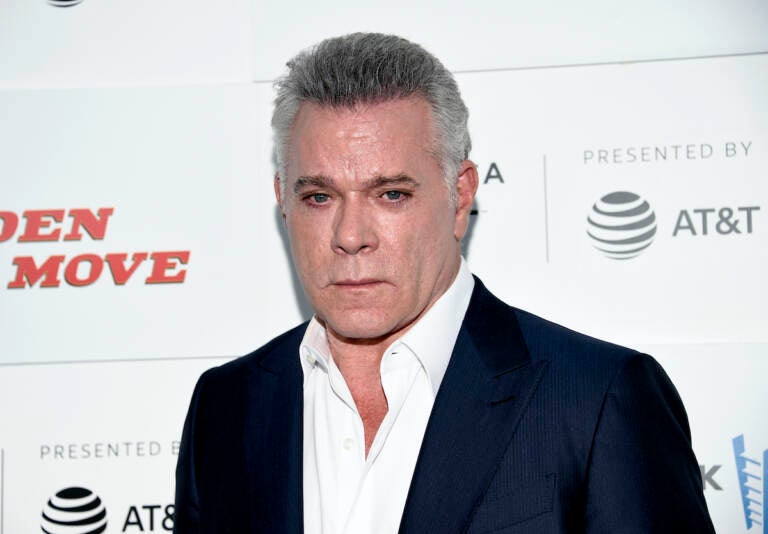In this celebrity appearance photo, Ray Liotta stands poised and slightly angled with his right shoulder back. He dons a dark navy-blue suit jacket over a white button-up shirt, casually unbuttoned at the top two buttons for a relaxed yet sophisticated look. His hair is a striking mix of dark gray on top and light gray on the sides, while his eyebrows remain a darker hue. His piercing dark blue eyes look directly at the camera, with his head subtly tilted downward.

The backdrop of the image is a white event board, partially obscured by Liotta himself. Visible segments of signage reveal logos and text, including "presented by AT&T," the AT&T globe, and fragments of other words like "DENMOVE" and "STAIRS," indicating a mix of event sponsors. The actor appears to be in his early 60s, attending what seems to be a formal event or a charity function.